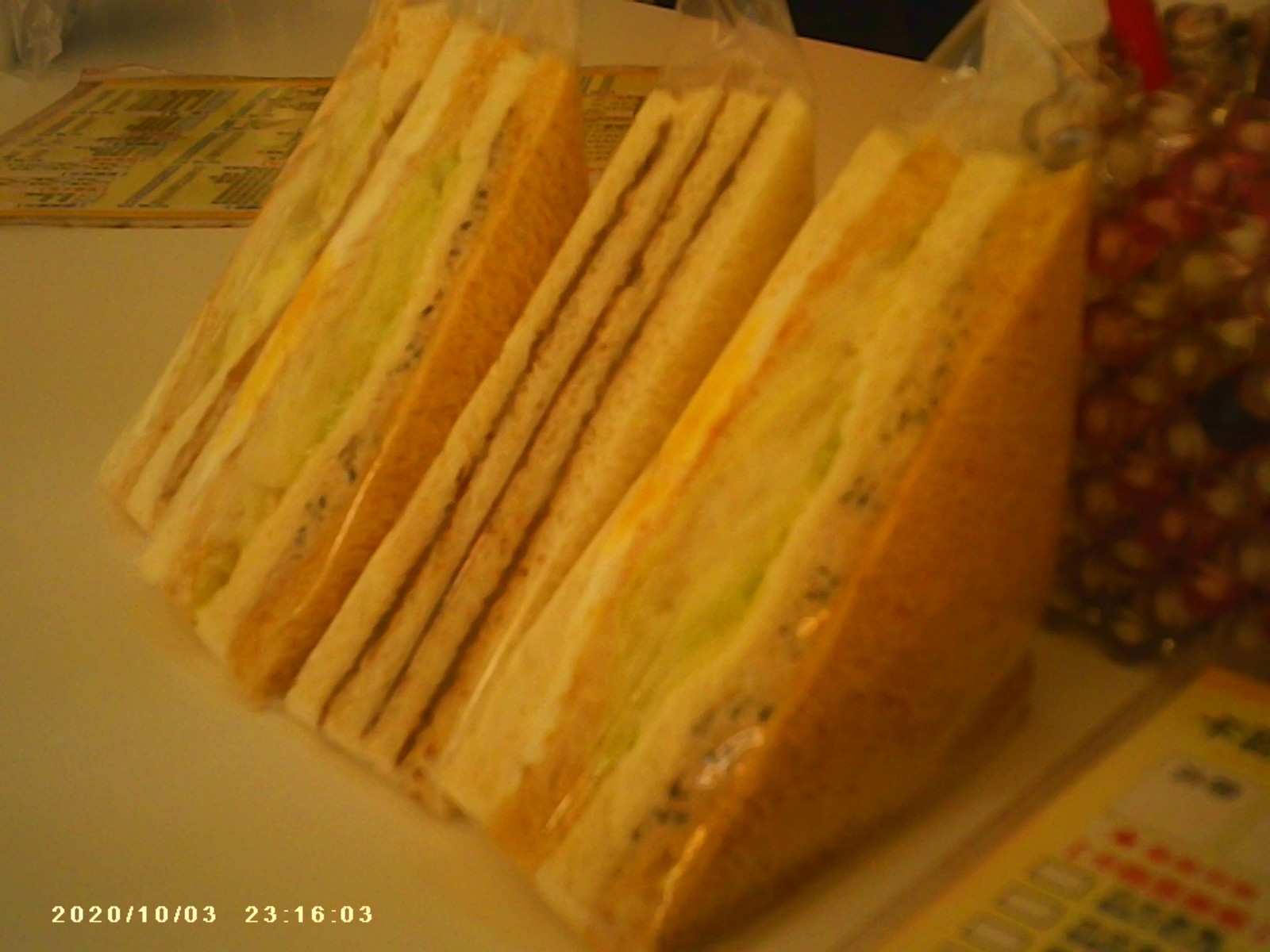In this digital photo dated October 3, 2020, at 23:16:03, three triangular cut sandwiches, each individually wrapped in plastic bags, are positioned upright on a white, laminated countertop, likely within a 7-Eleven or similar convenience store. The sandwich on the left and right both appear to be of the bacon, lettuce, and tomato variety, with visible lettuce and meat between the bread slices. The middle sandwich departs from this theme, featuring strips of bacon and possibly a thin spread of dark substance, potentially peanut butter or jam. Surrounding the sandwiches, the countertop holds additional objects, including what looks like restaurant menus or placemats, and a possibly olive-filled bottle. Noticeably, the image carries a yellowish filter, hinting at artificial lighting or an applied photo filter. The overall setting is slightly blurry, indicative of a casual snapshot capturing everyday convenience store offerings late at night.